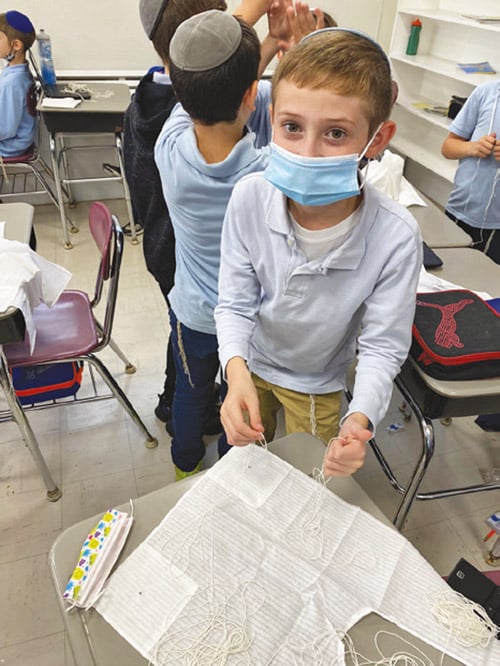In this vibrant classroom scene, a young boy with sandy hair and striking blue eyes gazes directly at the camera, his face partially obscured by a blue surgical mask, capturing a moment from the COVID-19 pandemic era. He wears a light blue shirt and beige slacks, and a medora rests on the back of his head. In his hands, he holds a piece of string, poised over a large sheet of paper on his desk, suggesting he might be crafting a kite. Surrounding him, more boys can be seen in the background, also wearing medoras and focused on their own projects, their desks similarly equipped with materials. The classroom is filled with small white desks and reddish chairs, indicative of an elementary school setting. Lunch bags and other classroom materials are scattered around, while some girls are seated by the windows, adding to the lively, collaborative atmosphere of the scene.